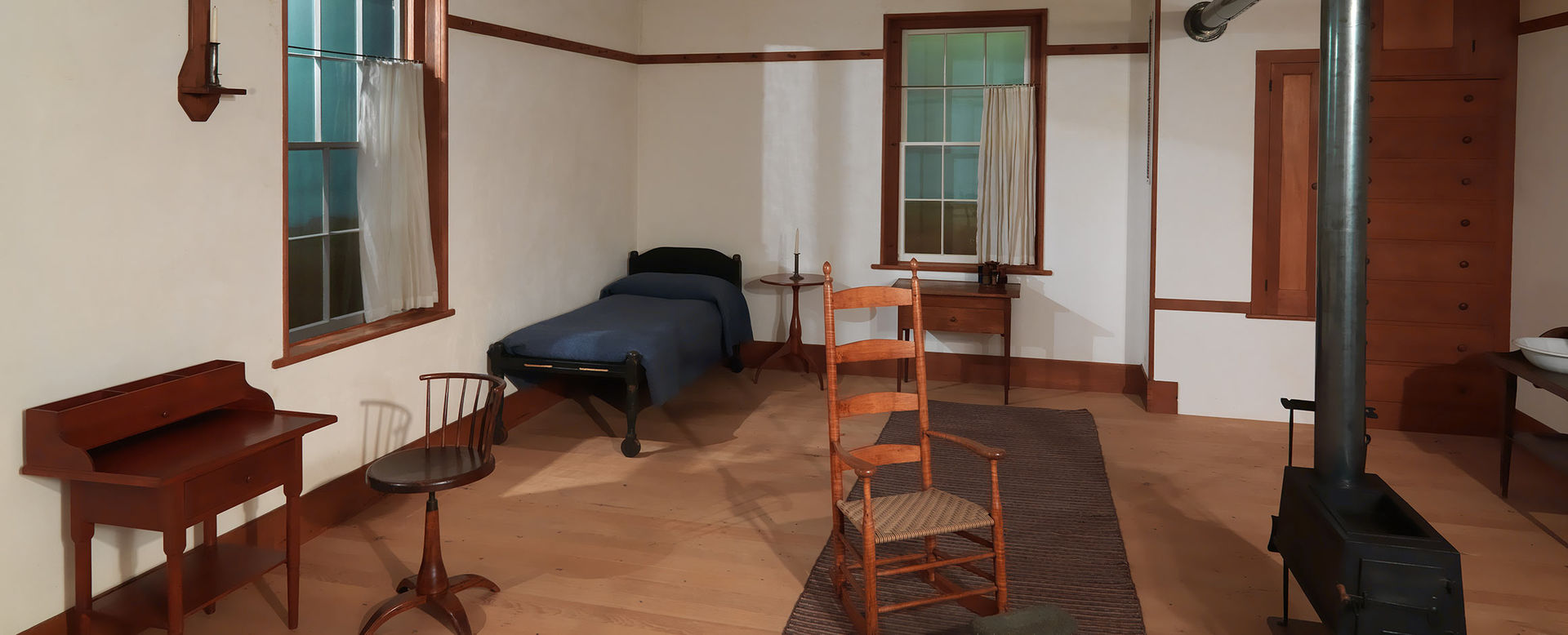This photograph captures the interior of a modest, minimalist bedroom, reminiscent of the turn of the century or even the 1800s. The room is characterized by white walls adorned with dark wooden windowsills, baseboards, and trim near the ceiling. Two large windows, one on the left and one at the back, are framed with dark wood and dressed with white curtains that cover three-quarters of the window height, leaving the tops unshielded. 

At the center back of the room, a black iron wood-burning stove, its cylindrical chimney rising and curving toward the rear wall for smoke expulsion, anchors the space. In front of the stove stands an old-style wooden chair. Beside it, there is a narrow, old-fashioned single bed, just wide enough for one person, featuring a headboard and solid legs, and draped with a blue blanket. Adjacent to the bed is a simple nightstand and a small table beneath the rear window.

An old wooden desk accompanied by a stool with a small back is placed in the left foreground of the room. Towards the right of the room, on the wall, a tall dresser, or some sort of storage unit, stands alongside a basin setup, indicative of a time when such items were used for washing hands and faces.

A narrow, rectangular rug stretches across the wooden floor, upon which sits a wooden rocking chair. The room's sparse yet functional furnishings highlight its utilitarian charm and evoke a sense of historical simplicity.